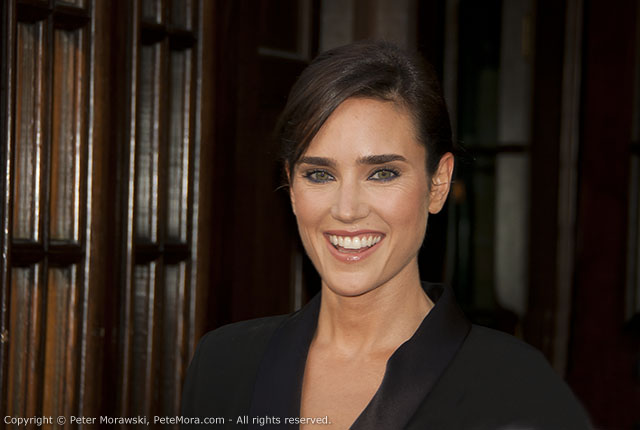This is a detailed photograph of an attractive young actress centered in the frame, sporting a radiant smile with her mouth slightly open. Her brunette hair is parted on the side and elegantly pulled back into an updo, complementing her hazel eyes accentuated by subtle eyeliner and likely a touch of lip gloss. She is dressed in a stylish black blouse or jacket, featuring slightly shinier lapels that add a touch of sophistication to her outfit. The backdrop consists of a dark brown wooden door with windows, providing a warm and classic contrast to her ensemble. At the bottom left-hand corner of the image, the text, "© Peter Morowski, PeteMora.com - All Rights Reserved," is clearly visible. The photograph exudes a professional quality, suggesting it could have been taken by paparazzi or a fan during an event, possibly a premiere, given her joyful demeanor and poised appearance.